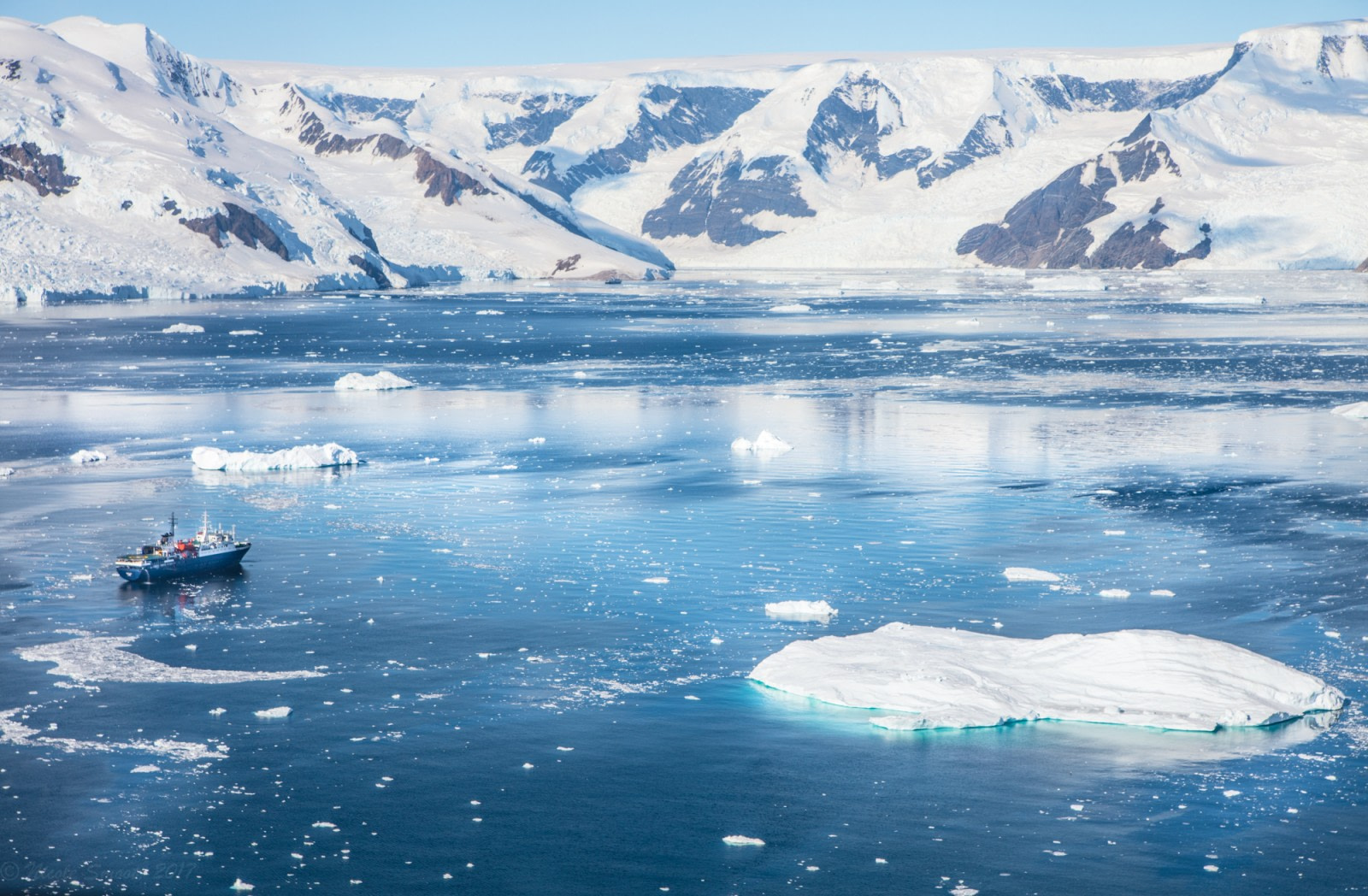The photograph showcases an icy, snow-laden landscape that evokes the stark, frigid beauty of polar regions. The scene features a broad expanse of ocean covered with sheets and chunks of ice, glistening with a cold, beautiful blue hue. In the midst of this harsh, frozen seascape, a lone cargo ship navigates through the icy waters, its purpose unclear but suggesting a voyage of exploration or transport.

Beyond the ice-filled ocean, the upper portion of the image reveals rugged, mountainous terrain, with rocky faces cloaked in thick blankets of snow and ice. These snow-capped mountains and hills further accentuate the severe, wintry environment. The sky above is pale and overcast, contributing to the overall cold and desolate atmosphere of the scene.

While the exact location of this landscape remains ambiguous, it could plausibly be somewhere within the Arctic, Antarctica, or even high latitude regions like Greenland, northern Canada, or Norway. The photo captures the essence of an environment shaped by intense cold and significant snowfall, conveying the formidable, yet captivating, nature of such remote places.